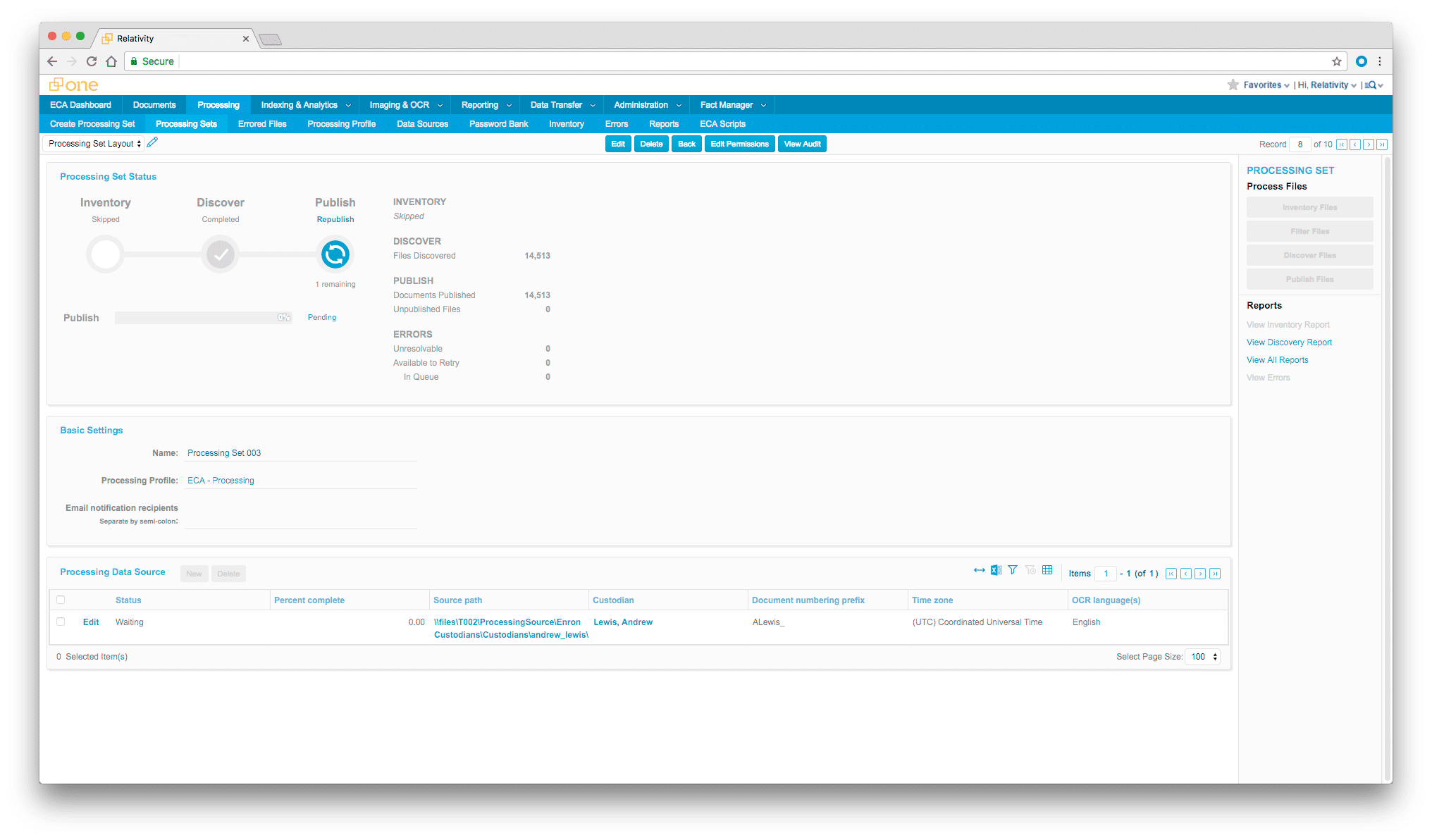The image depicts a labeled webpage interface with distinguishable elements. In the upper left-hand corner, there is a tab featuring three circular buttons: a red circle, a yellow circle, and a green circle. Just below the tab, an address bar is situated, which is currently empty. To the left of the address bar, there is a black left-pointing arrow (the back button) and a gray right-pointing arrow (the forward button). Adjacent to these arrows are a refresh button and a Home button.

Further down, '1' is prominently displayed in yellow font. Nearby, a logo consisting of two overlapping squares at their corners is visible. The overall design includes a blue horizontal menu bar extending across the page from left to right.